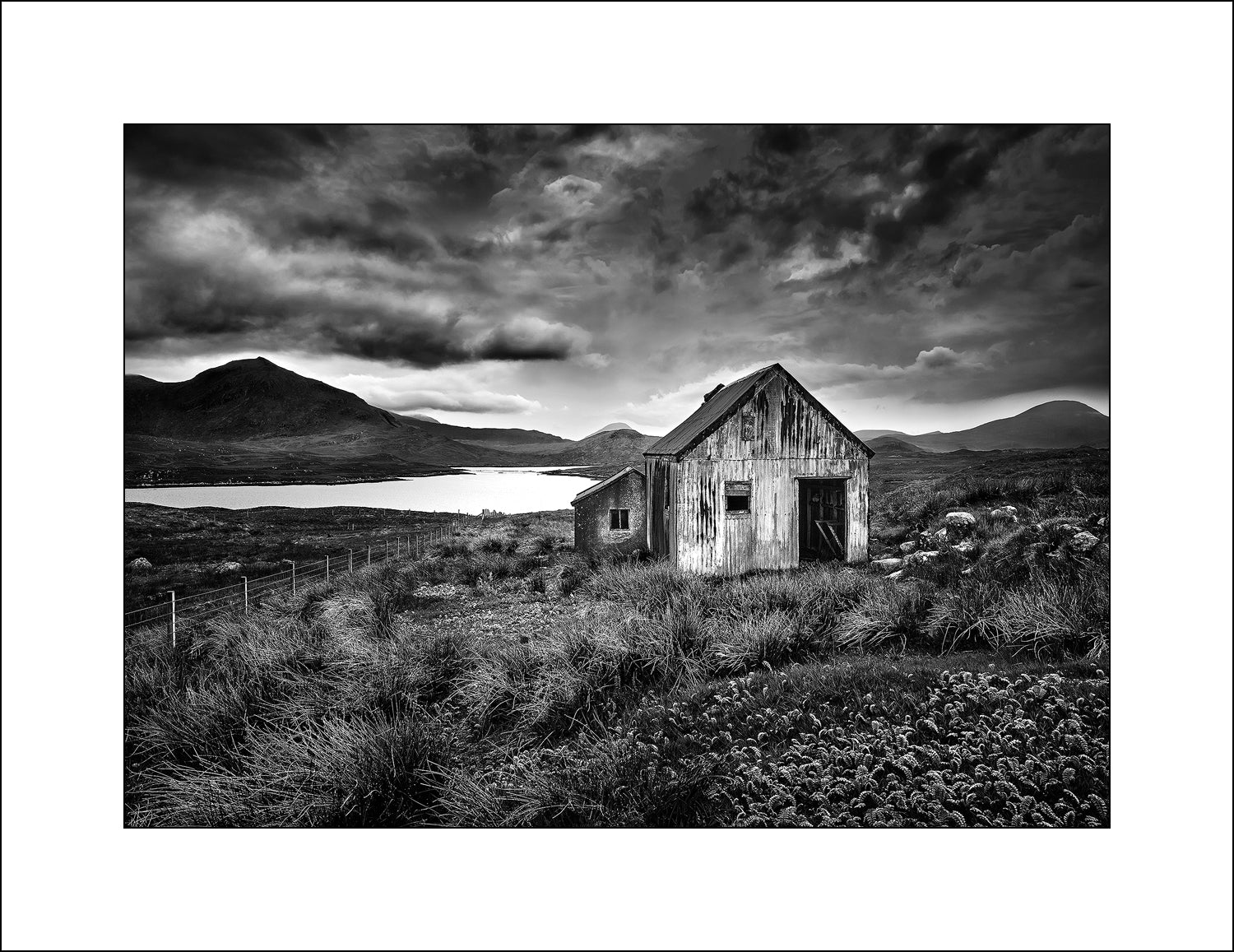This highly stylized black-and-white photograph captures a deeply atmospheric scene featuring a weathered barn standing in the middle of an overgrown, grassy field. While the barn, appearing as a two-story structure with an old, faded, almost peeling white paint, serves as the focal point, the photograph also portrays a powerful natural backdrop. Above the barn, dark storm clouds gather, lending a dramatic, moody ambiance to the image, suggesting an approaching or dissipating storm.

In the background, we can see the looming silhouette of a mountain peak, flanked by additional mountain ranges, adding a sense of depth and isolation to the scene. Nestled at the base of these mountains is a lake, further enhancing the quiet desolation. To the side of the barn, a small, barely visible road and thin electric poles are depicted, underscoring the remoteness and abandoned feeling of the place.

Enhancing the sense of antiquity and abandonment, the barn seems to have an extension on the side, possibly a smaller room or offshoot cabin, adding complexity to the structure. A thin wire fence stretches into the distance, adding to the feeling of seclusion. The overall saturation of the black-and-white tones is rich and deep, possibly digitally altered, intensifying the photograph's haunting and almost frightening mood. The photograph evokes a strong sense of isolation, as if it captures a forgotten place lost to time and nature.